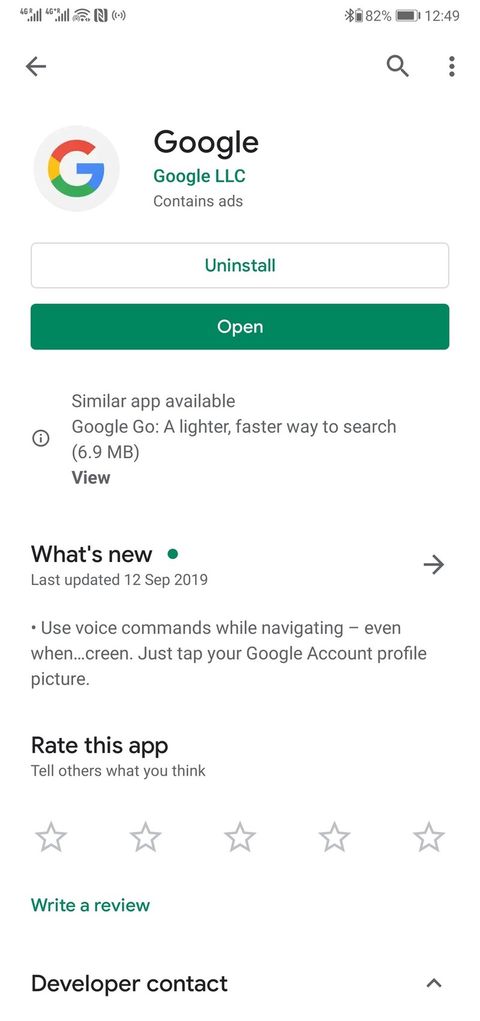In this image, we see a screenshot of a Google application interface on a cell phone. At the top of the screen, the status bar displays the phone’s signal strength, Wi-Fi connection, battery level, and clock. Right below this, the Google logo is prominently displayed alongside the text "Google LLC" and a note indicating that the app contains ads.

Further down, a white button with green font reading "Uninstall" is visible, followed by a green button with white text that says "Open." Below these buttons, there's a suggestion for a similar app: "Google Go, a lighter, faster way to search," which has a size of 6.9 megabytes and an option to view more details.

The section under "What's New" indicates the last update was on 12 September 2019, with an arrow pointing to the right for more details. The text below highlights new features, mentioning the ability to use voice commands while navigating even when the screen is off, prompted by tapping the Google account profile picture.

Lastly, there is a section prompting users to rate the app with five stars, write a review, and access developer contact information.